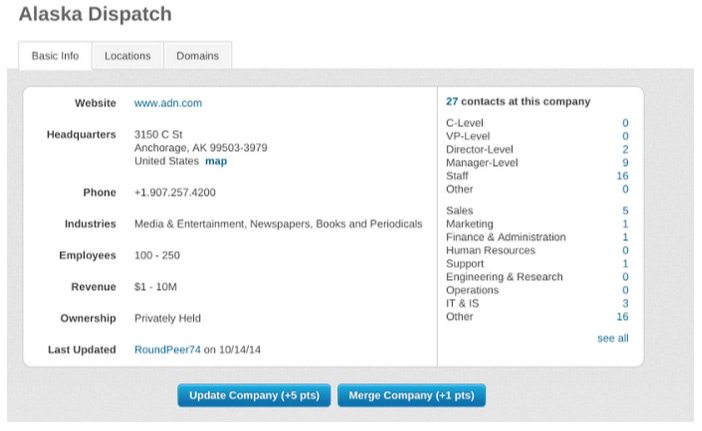In the upper left corner of the page, the header "Alaska Dispatch" is displayed in grey. Adjacent to it, there are three tabs labeled "Basic Info," "Locations," and "Domains," each enclosed by grey borders. The "Basic Info" tab is highlighted in white, indicating its active status. Below these tabs, a grey box contains a smaller white box displaying essential company information.

The details include the website URL "www.adn.com," the headquarters address "3150 C Street, Anchorage, Alaska, AK 99503-3979, United States," and a blue button that links to a map. Contact information includes a phone number, and the industries listed are "Media and Entertainment," "Newspapers, Books, and Periodicals."

Further specifics shown are the number of employees, the company's revenue, and its ownership status, which is "Privately Held." The page mentions the "Last Updated" date as well.

On the right side of the page, there is a detailed chart listing "27 contacts at this company," categorized by roles and departments. These categories include C-Level, VP-Level, Director-Level, Manager-Level, Staff, Other, Sales, Marketing, Finance and Administration, Human Resources, Support, Engineering and Research, Operations, ITIS, and Other, each accompanied by respective numbers.

At the bottom of the page, two blue buttons are present. The left button labeled "Update Company, plus five points" and the right button labeled "Merge Company, plus one point."